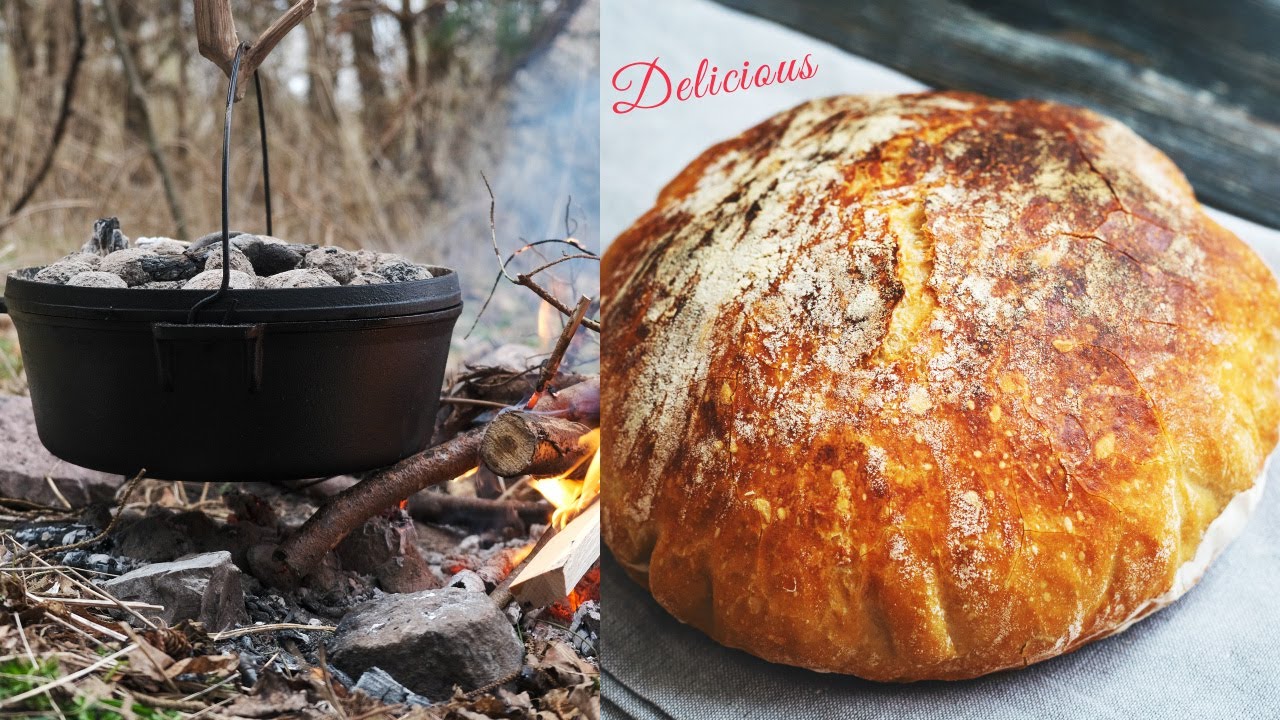This image is a collage composed of two square photos set side by side. The left photograph captures an outdoor scene with a cast iron pot hanging from a tree branch. The pot, featuring a black handle, is filled with small, round rocks or pieces of charcoal and is situated above a bundle of sticks, with an emerging flame on the right side suggesting a recently started fire. The background includes blurry tree branches and elements of a rustic outdoor setting, such as stones, dirt, and twigs.

Contrasting this, the right photograph showcases a delectable round loaf of bread with a beautifully baked, toasted crust. The crust varies in color from dark brown on top to beige and tan on the edges, with a dusting of white flour and some cracks revealing the bread's interior. This loaf rests on a light gray folded cloth. To the top left corner of this image, the word "Delicious" is displayed in a stylish red cursive font, diagonally enhancing the visual appeal of the scene. Together, these images evoke a sense of rustic cooking and artisan baking.